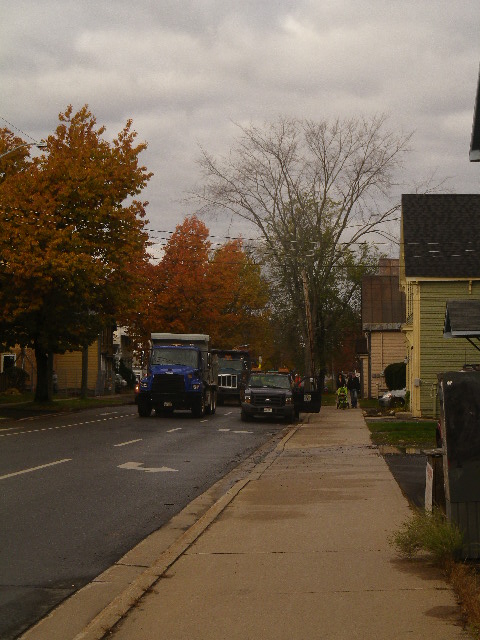This photograph depicts a city street scene on an overcast day, capturing a vivid tableau of fall with various shades of yellow, orange, and green in the trees lining the road. On the right, a wide light brown cement sidewalk borders a neon yellow wooden house with a black roof, alongside a tan house with a brown roof. Further down the street, a house nearly out of view has a gray roof. Trees on the right are partly green with one being completely bare, while those on the left range from light brown to vibrant orange and light green. 

The black paved road features white lines, a right-turn arrow, and several trucks: a dark blue truck with a gray bed, a black dump truck, and a regular-sized black pickup truck with its door open. Vehicles appear on the left side of the street, moving towards the camera, suggesting it may be a one-way road or a region where vehicles drive on the opposite side. Additionally, two individuals, one possibly pushing a stroller, can be seen walking on the sidewalk, adding a touch of life to this autumnal urban landscape.